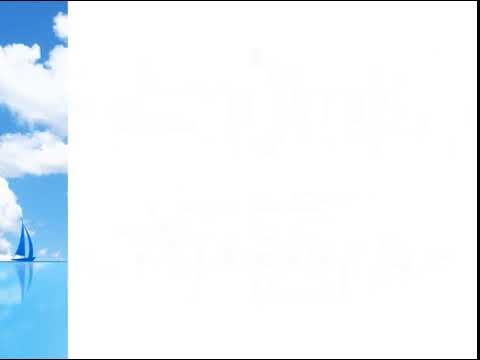The image is a square composition. On the left side, there is a very narrow vertical strip showing a serene scene: a glassy blue body of water with a blue sailboat resting on the horizon, creating a pristine reflection in the water. Above this tranquil setting is a vibrant blue sky adorned with puffy white clouds, which are also mirrored in the water below. The rest of the image is a stark, solid white background that fills the remainder of the square. The white area is bordered by thin black lines at the top and bottom, and a thicker black line runs down the right side, connecting the two thinner lines. Notably, the left side where the vertical strip of sky, water, and sailboat is depicted, remains unbordered, further emphasizing the minimal but detailed and picturesque scene captured in the strip.